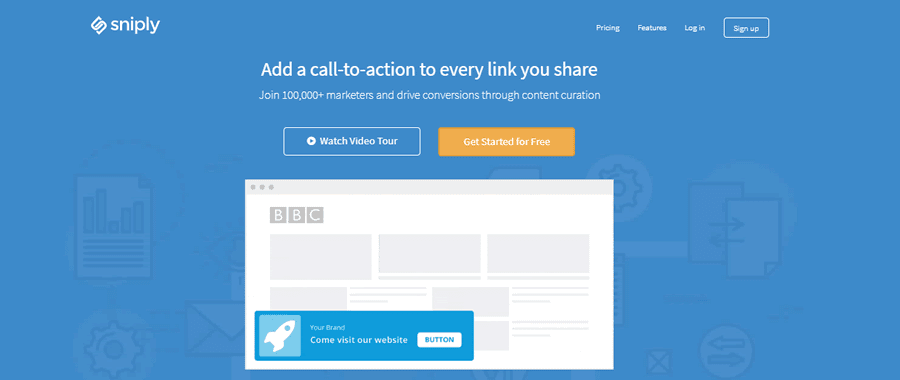The image depicts a sleek and modern website with a gradient background transitioning from white to medium blue. On the upper left side, there is a distinctive logo featuring the letter 'S,' which is creatively intertwined with two 'U's, followed by the word "Snipply" in white text. 

Positioned towards the top right, there is a navigation menu with the options "Pricing," "Features," "Login," and "Sign Up," all capitalized, with "Sign Up" enclosed in a square for emphasis.

Centrally placed, a prominent header in large white font reads, "Add a Call-to-Action to Every Link You Share," with hyphens connecting the phrase for clarity. Beneath this, a subheader invites users to "Join 100,000+ marketers and drive conversions through content curation."

Below the main text, a white-bordered button with the label "Watch Video Tour" in white print is prominently displayed. Adjacent, a yellow-orange banner encourages users to "Get Started for Free."

Further down the page, a section features a square with a gray banner at the top and the BBC logo underneath. At the bottom, a blue rectangle matches the background hue, displaying a square icon of a diagonally ascending rocket with the text "Your Brand, Come Visit Our Website." Additionally, there is a white button with the word "Button" inscribed in blue print.